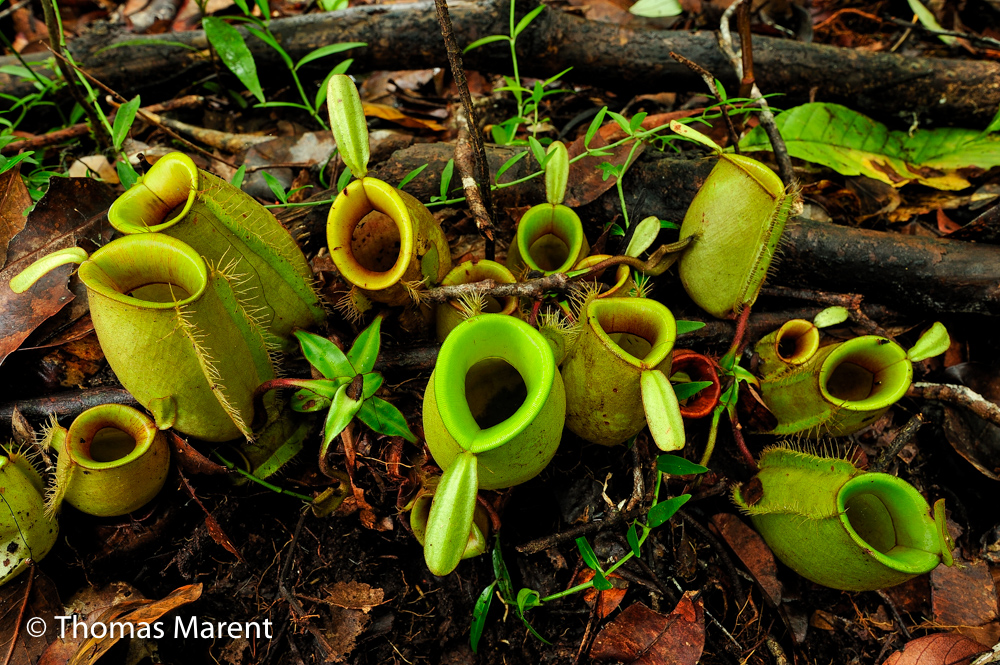This vibrant, color-edited photograph, taken by Thomas Merent, portrays an almost ethereal scene on the forest floor with a cluster of approximately ten bright green pitcher plants. Each pitcher plant is flask-shaped with an oval opening at the top and extensions resembling handles near the upper portion. Some of the plants display hairy spines on their sides. The pitchers come in shades of lime green, bright green, and golden, creating a striking contrast against the wet, brown leaf-littered ground. The soil appears saturated, possibly from a recent rain, adding a glossy sheen to the fallen leaves, tree logs, and scattered green shoots that resemble vines or grasses. The open lids of the pitcher plants allow a glimpse inside where water or sap is visible, highlighting their carnivorous nature in this lush, forested environment. The scene is captured in landscape orientation from a standing perspective, showcasing the rich detail and realism of the photographic representational style.